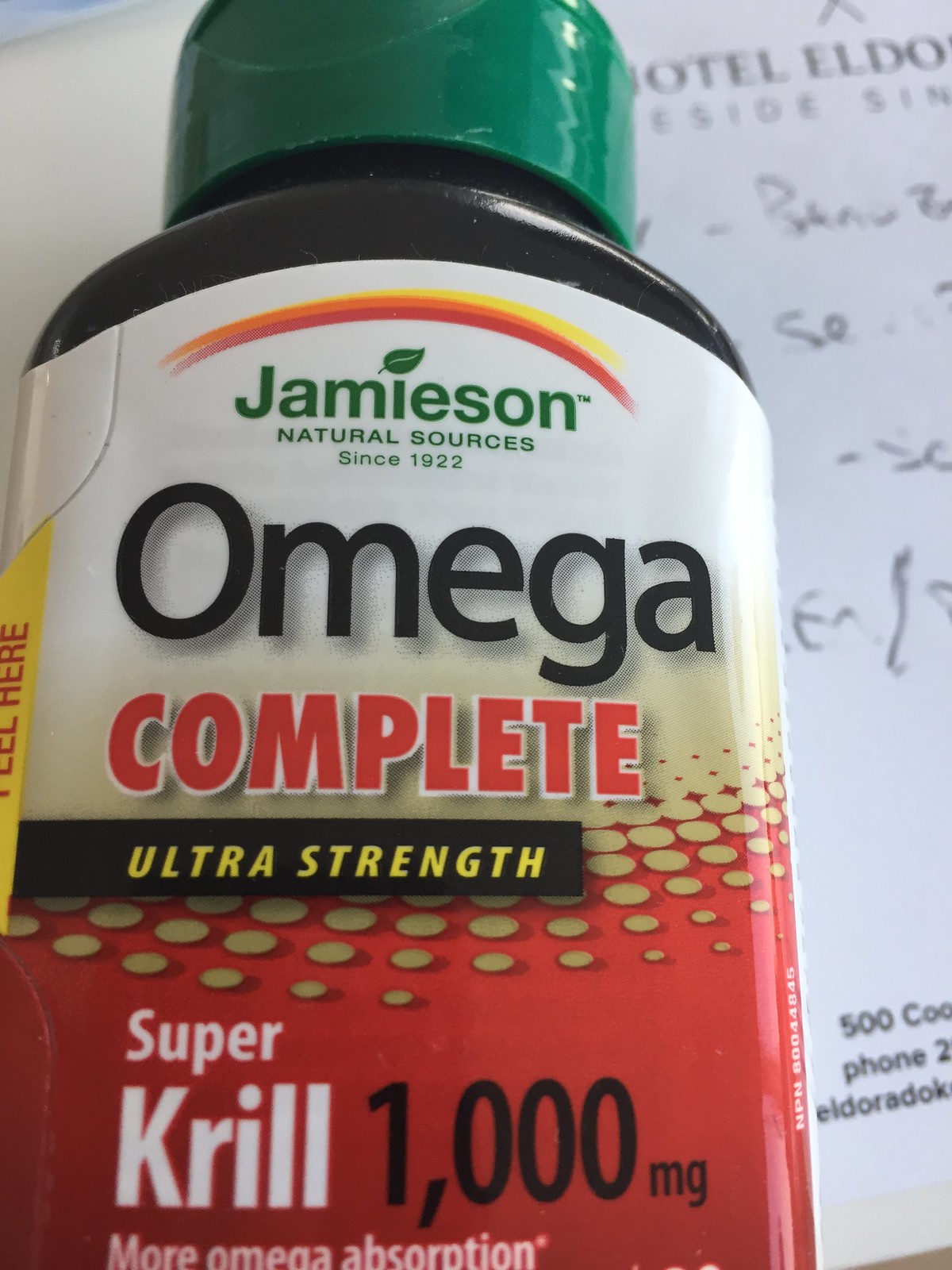This is an extreme close-up photograph of a dietary supplement bottle taken indoors. The bottle is about six inches tall and four inches wide, predominantly black with a forest green cap. The label is intricate and divided into distinct sections with different colors and typography. 

Starting from the top, the label features a white background with a small yellow, orange, and red rainbow icon. Just below this, in green text, it reads "Jamieson Natural Sources since 1922," with the dot over the 'i' designed as a leaf. The middle section of the label prominently displays the word "Omega" in large black font, followed by "Complete" in red font. Separating these sections is a black banner with gold text reading "Ultra Strength."

The bottom half of the label transitions into a red background with a light tan or khaki halftone pattern overlapping it. Within this section, "Super Krill" is boldly printed in white, while "More Omega Absorption" appears in smaller white text underneath. Finally, "1000 MG" is stated in black font. Behind the bottle, a white piece of paper is visible with the words "Hotel Eldo" on it.